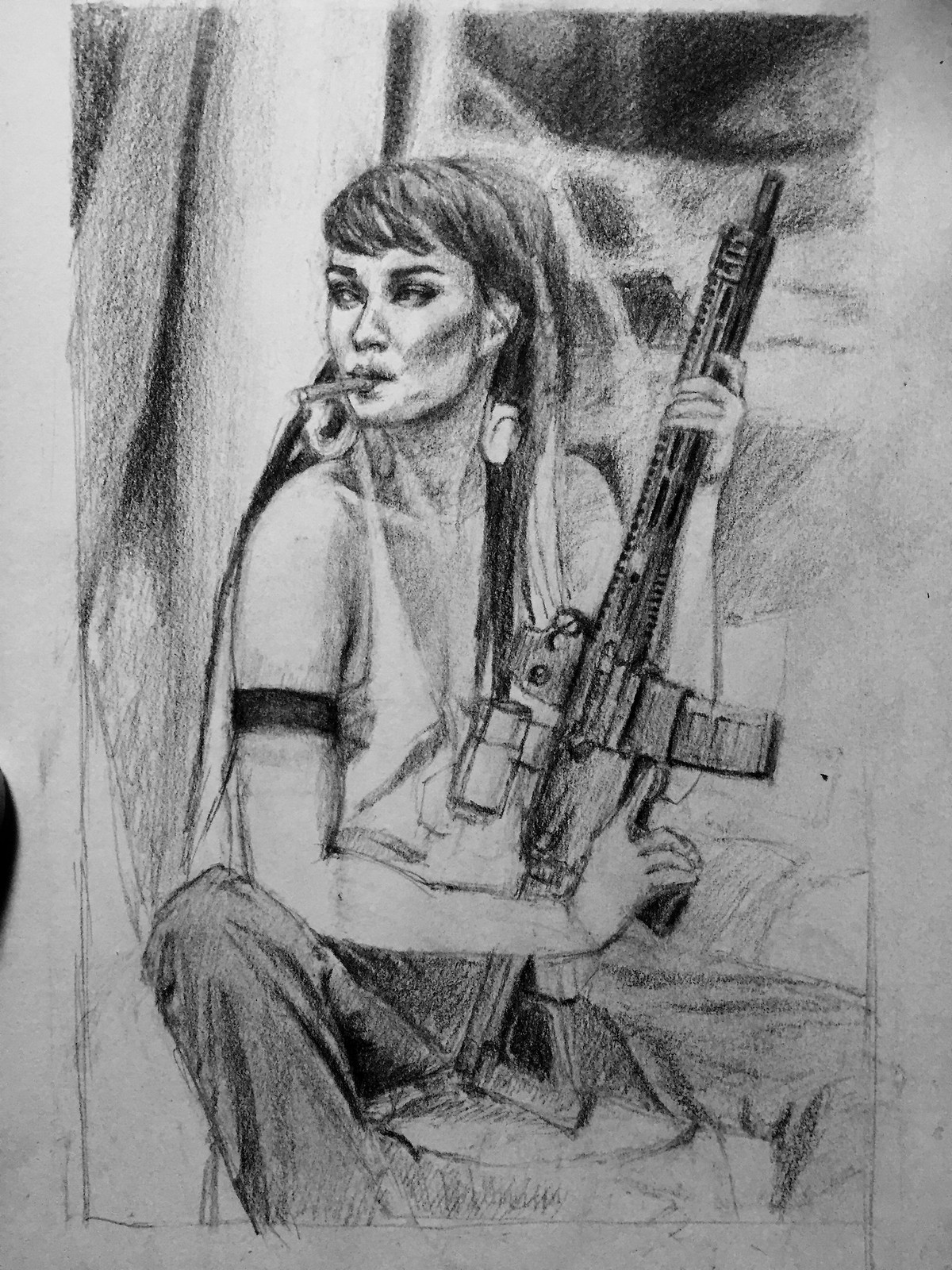This is a detailed photograph of a charcoal drawing on a piece of paper, depicting a woman holding an automatic firearm. She is seated in a stairway or alcove, projecting a sense of contemplation and resolve. A cigarette dangles from her lips as she gazes off-camera to the left, her expression enigmatically defined through subtle shading. The artwork predominantly uses shades of black, white, and grayscale to convey depth and emotion. The drawing is semi-realistic; while it captures the essence and posture of the woman with a photographic quality, it lacks fine details like fingernails and eyelashes, leaving these elements to the viewer's imagination.